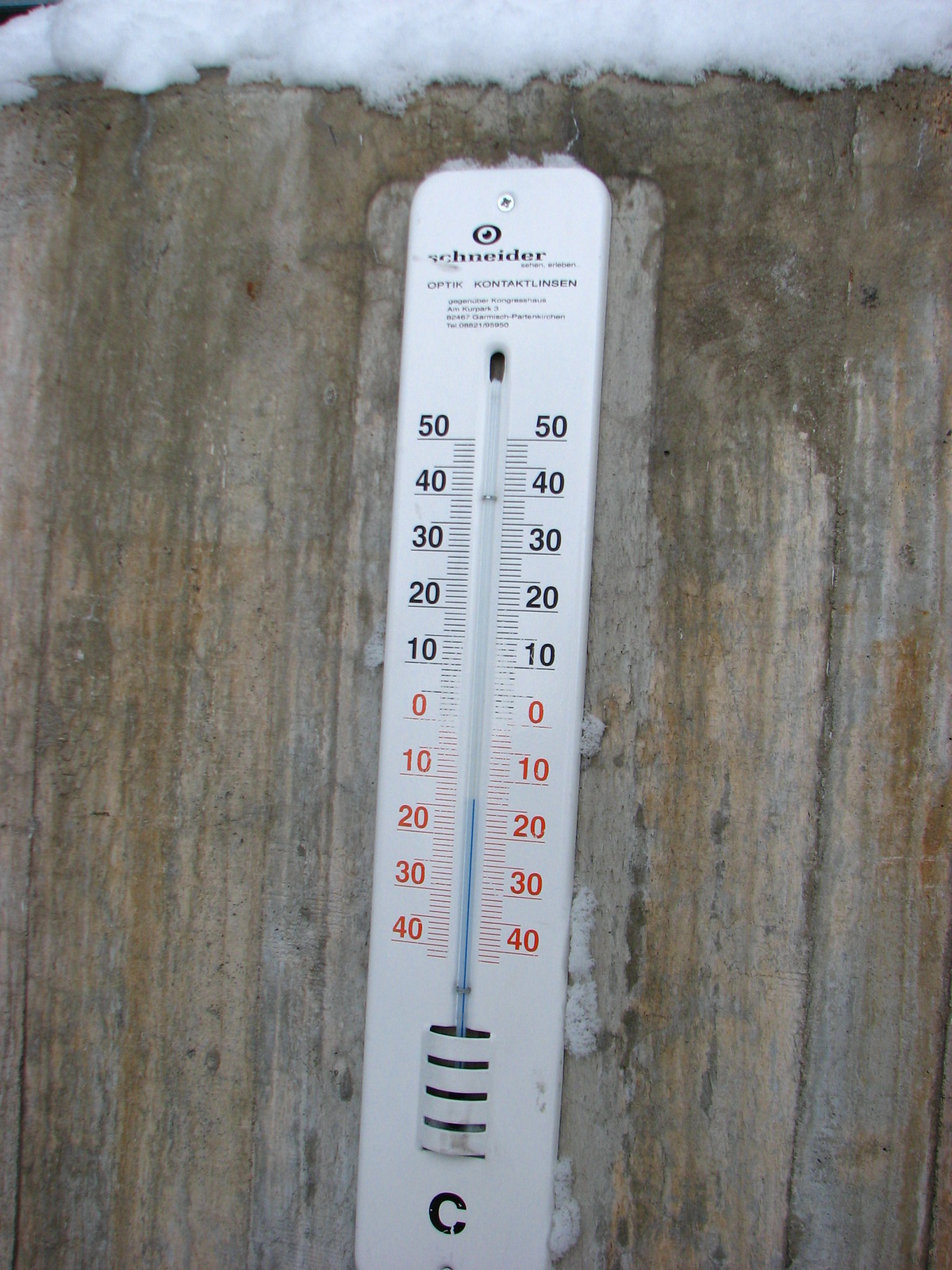The image features a close-up view of a newly installed Schneider thermometer affixed to a tree trunk. The thermometer is securely screwed into the tree at the top. Traces of an older thermometer's outline are visible, suggesting a replacement. The tree trunk displays a rich texture with varying hues, ranging from darker wood to lighter, washed-out areas with touches of tan. Atop the trunk, about an inch of snow rests, adding a wintry atmosphere to the scene.

The thermometer showcases two sets of numbers: the black numbers range from 50 to 10 in descending order, while the red numbers span from 0 to 40. A large "C" is visible near the bottom, indicating that the measurements are likely in Celsius. The glass tube of the thermometer, highlighted in blue, covers a temperature range from -40 to 50. The image captures the intricate details of both the thermometer and the tree trunk, offering a vivid snapshot of an outdoor winter environment.